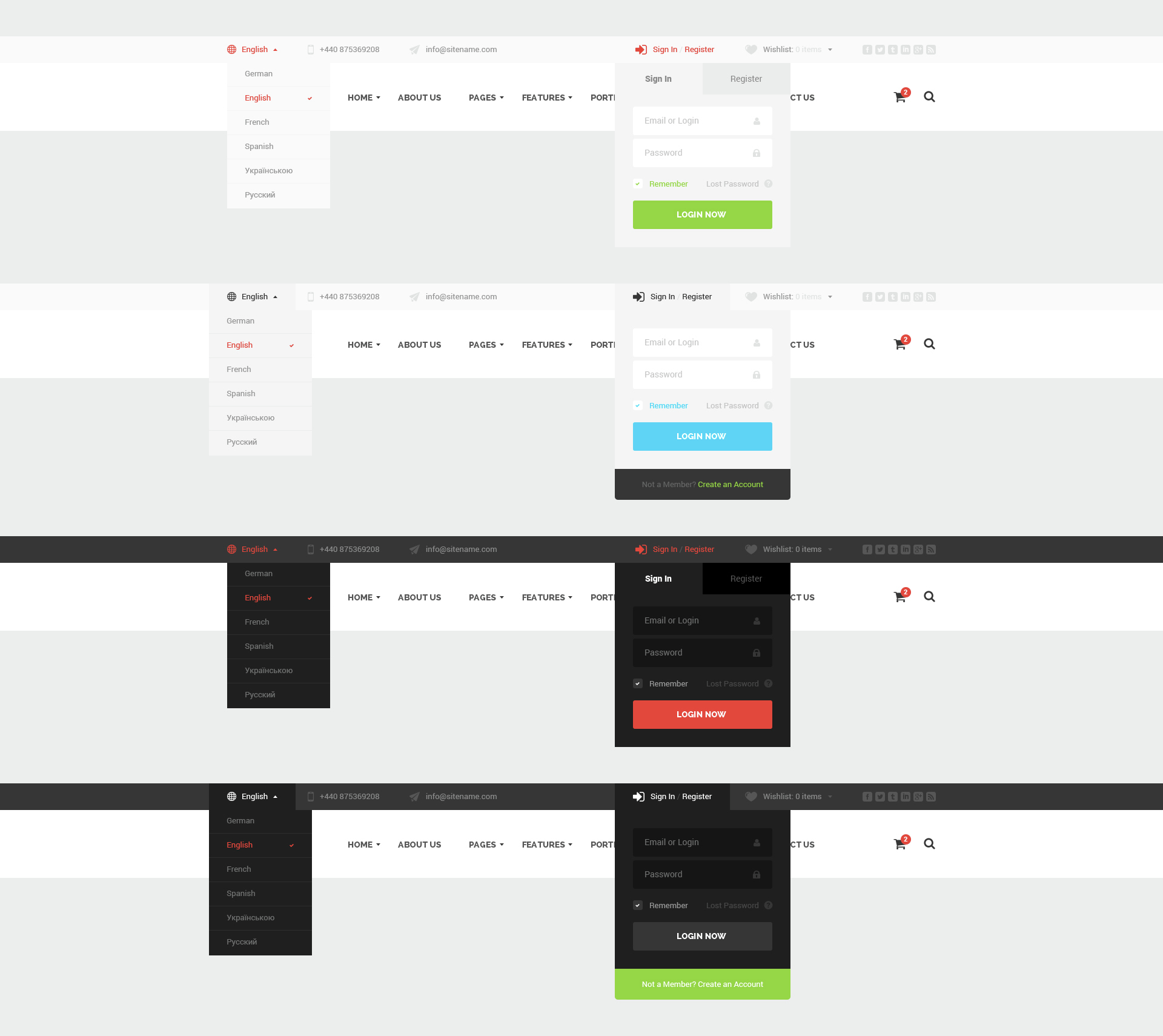The digital image showcases a multilingual website interface with language options for English, German, French, and Spanish. The navigation menu includes links to the Home page, About Us sections, and various Features. A prominent pop-up window urges users to "Log In Now," while a small shopping cart icon in the upper-right corner indicates 2 items. The language selection row shows that English is currently selected. Additionally, users have the option to create an account. Contact information is provided at the bottom, featuring an email address (info@sitename.com) and a phone number (+44 0-753-69208).